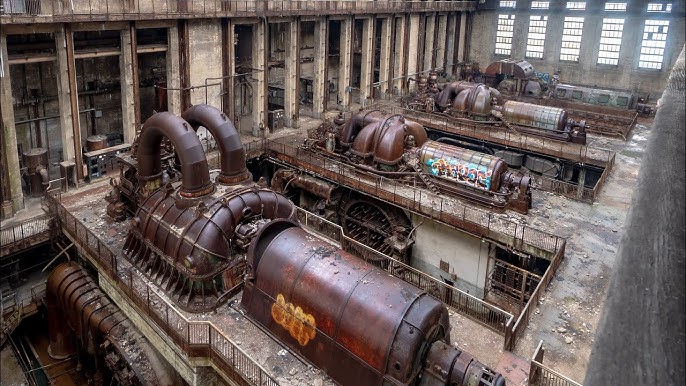The photograph captures an elevated, overhead view of an old, abandoned factory interior. The facility is dominated by several large, dark brown, metal machinery stations that resemble generators or engine-like structures, complete with extensive metal tubing. These machines, positioned on concrete flooring surrounded by metal railings, show signs of rust and are covered in random graffiti, suggesting a long period of disrepair. Notably, there is visible graffiti, including a stylized "D-O-I-R" at the bottom right and blue, blurry text in the center. The factory features concrete pillars and a stone-colored light beige wall in the background. Bright sunlight streams through five large windows located in the upper right corner, casting ample light over the scene. Rubble strewn across the floor and the general dirtiness further emphasize the facility's neglected state.